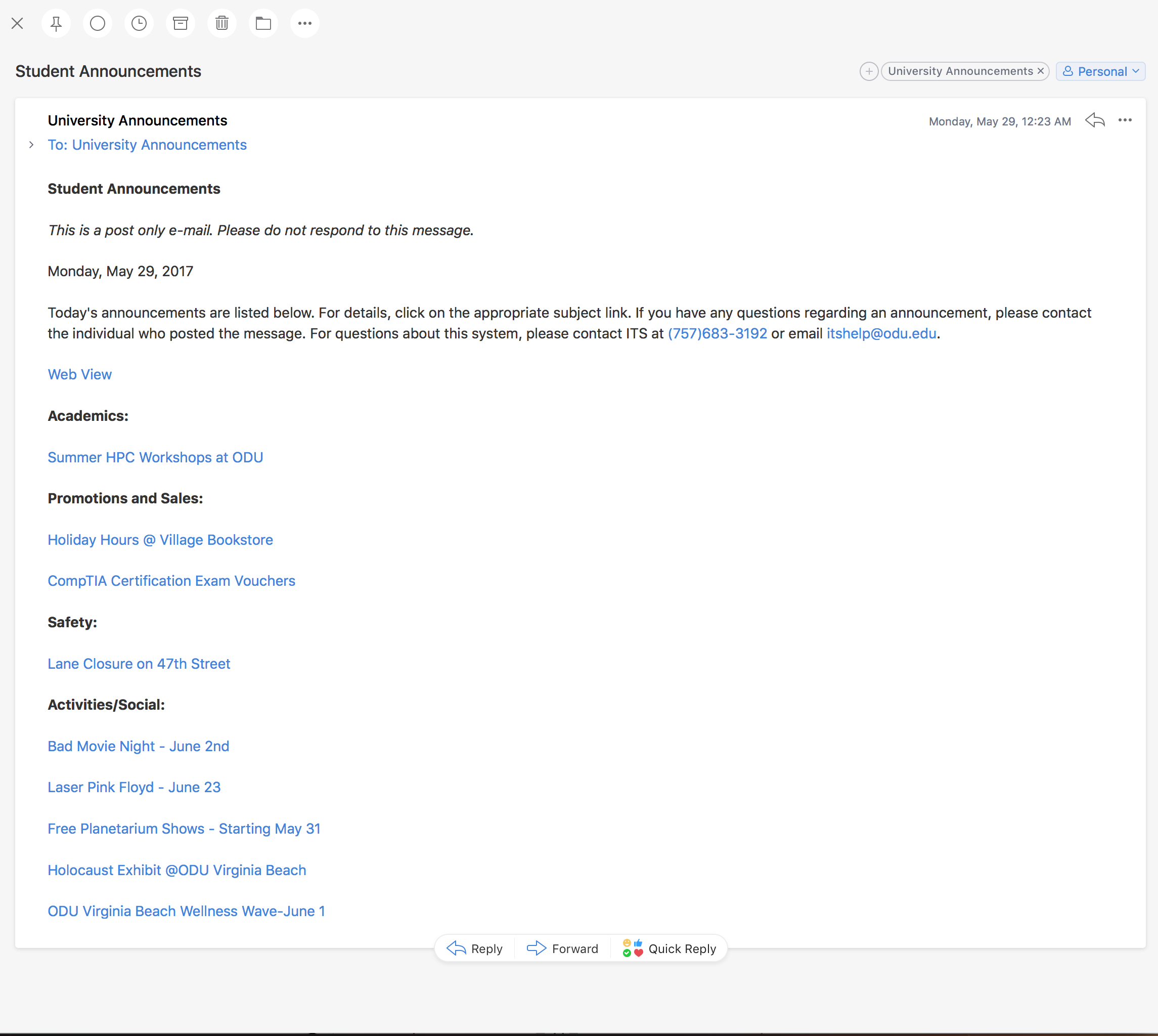**Screenshot of University Announcement Webpage**

The image captures a screenshot of a university announcement webpage, featuring a clean and organized layout underscored by neutral background elements. 

**Top Section:**
- The uppermost part of the page is framed by a gray bar, which spans the entire width. 
- In the top left corner, a small "X" icon is visible, allowing users to close the page.
- Just right of the "X" icon, there's a sequence of circular icons each with distinct functionalities:
  - A pushpin icon, signifying a pinned item.
  - A circular icon, which could denote a refresh or reload function.
  - A clock icon, likely indicating recent or timed occurrences.
  - A filing cabinet icon, probably for archived items.
  - A trash can icon, meant for deleting items.
  - A folder icon, representing file organization.
  - Three horizontal black dots, suggesting an overflow menu for additional options.

**Main Content Area:**
- Positioned towards the top right corner of the content area, there is an oval with black text that reads "University Announcements."
- Adjacent to this, there is a blue square labeled "Personal" – potentially a category or a user-specific section.

Beneath these elements, the main body of the page displays a detailed announcement:
- A prominent heading with black font states "University Announcements."
- Below the heading, there is a hyperlinked text that directs users to the "University Announcements" page for further details.
- Following this, another section is labeled as "Student Announcements" with the text specifying: 
  - "This post only email. Please do not respond."
  - Dated "Monday, May 29, 2017."
  - A brief introduction to the announcements for the day: "Today's announcements are listed below. For details, click on the appropriate subject link."
  - An advisory note: "If you have any questions regarding an announcement, please contact the individual who posted the message."
  - A technical support reference: "For questions about this system, please contact ITS at 757-683-3192."

**Bottom Section:**
- Completing the layout, another horizontal gray bar runs along the bottom of the page.
- Beneath this, a thin black line serves as a subtle footer demarcation, reinforcing the structured design.